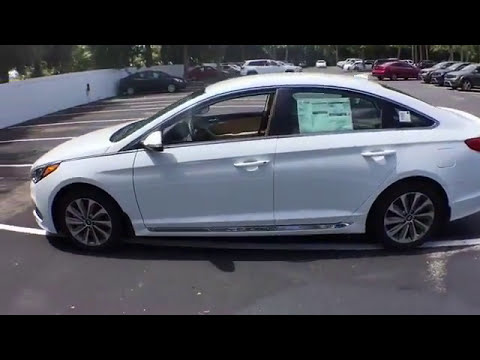In this image, a bustling parking lot stretches across the scene under daylight. The foreground prominently features a white, four-door sedan, distinguished by dealership information posted in its back window, suggesting it may be new or for sale. This car, which includes visible rims and an open driver's window, is haphazardly parked in an elongated spot capable of accommodating almost two vehicles, its position slightly askew from the designated lines. Surrounding the foreground car, numerous vehicles are systematically backed into their spaces. Enclosing the parking lot on the left is a white concrete wall, about waist-high, beyond which a grove of green trees is visible. The background is densely populated with more cars and additional trees scattered throughout, enhancing the sense of a vibrant and active location. The gray asphalt of the parking lot indicates a typical urban or suburban setting.